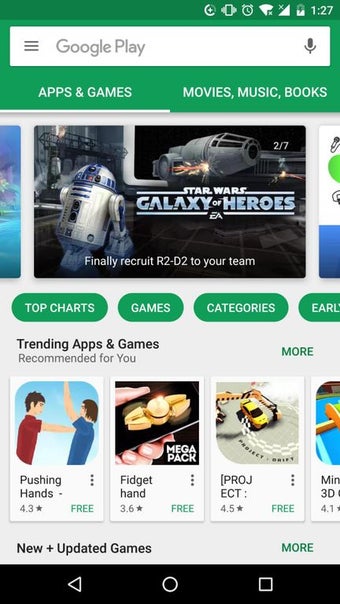This screenshot depicts the Google Play Store interface on an Android smartphone. The interface is characterized by a striking green gradient bar at the top of the screen, transitioning from dark green on the left to light green on the right. 

In the upper-right corner of this bar, various status icons are displayed: a fully filled WiFi symbol, fully filled cellular bars with an "X" to the left, indicating no cell service, and a half-charged battery icon displaying a charge symbol in the middle with the numeric indicator reading "127".

Directly below this bar is a white search box featuring three horizontal lines stacked vertically (the menu icon) on the left, with "Google Play" text adjacent to it. On the far right of this box, there is a grey microphone icon.

Under this search box, there are two main categories written in white font: "Apps & games" and "Movies, music, books," with "Apps & games" currently selected. A white underline indicates the selected category.

Below these categories, a prominent tile for the game "Star Wars: Galaxy of Heroes" is displayed, annotated as "2 of 7". Below this are green horizontal navigation bubbles labeled "Top charts," "Games," "Categories," and a partially cut-off bubble showing the word "Early."

Further down, the interface showcases sections labeled "Trending apps & games" followed by "Recommended for you," displaying a partial view of four recommended games. The rightmost game’s tile is partially cut off, but there is an option labeled "More" at the top-right corner, inviting users to explore additional recommendations.